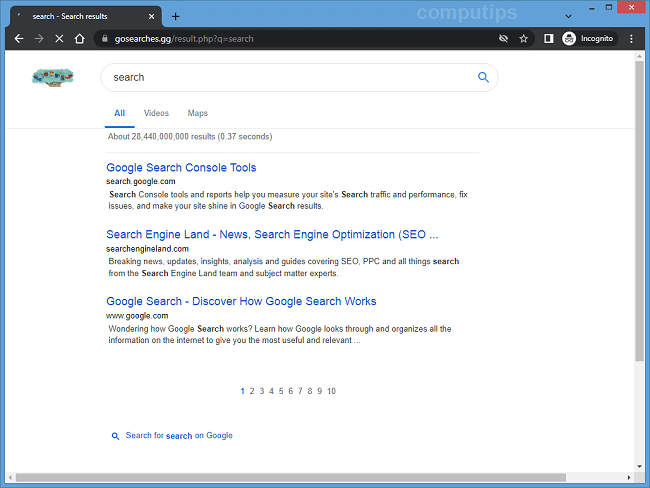Here is the cleaned and detailed caption:

---

This image showcases a search results page from a website. In the top-left corner, a browser tab displays "Search Results" in white text on a black background. To the right, there is a black "X" icon, a downward-facing arrow, a minimize icon, and a close tab icon highlighted in red.

Below the tab bar, a cartoon tree with green leaves and a brown trunk is visible on the left side. To its right, there is a search bar containing the word "Search" in black text.

Directly underneath, there is a navigation bar with options: "All" in blue and underlined, "Videos" and "Maps" both in gray. Below this, on the left, is text indicating "About 28,440,000,000 results in 0.37 seconds."

The main section of the search results lists are as follows:

1. "Google Search Console tools" in blue, followed by "search.google.com" in black. A description underneath reads: "Search Console tools and reports help you measure your site's search traffic and performance, fix issues, and make your site shine in Google search results."

2. "Search Engine Land – News, Search Engine Optimization (SEO)" in blue, with "searchengineland.com" in bold black. The description states: "Breaking news, updates, insights, analysis, and guides covering SEO, PPC, and all things search from the Search Engine Land team and subject matter experts."

3. "Google Search - Discover How Google Search Works" in blue, linked to "www.google.com." Below this, it says: "Wondering how Google Search works? Learn how Google looks through and organizes all the information on the internet to give you the most useful and relevant..." with ellipsis indicating a continuation.

At the bottom of the page, pagination options from 1 to 10 are available, with the number 1 highlighted in blue. Further down and to the left, there is another search bar with a magnifying glass icon and the prompt "Search first search on Google" in blue text.